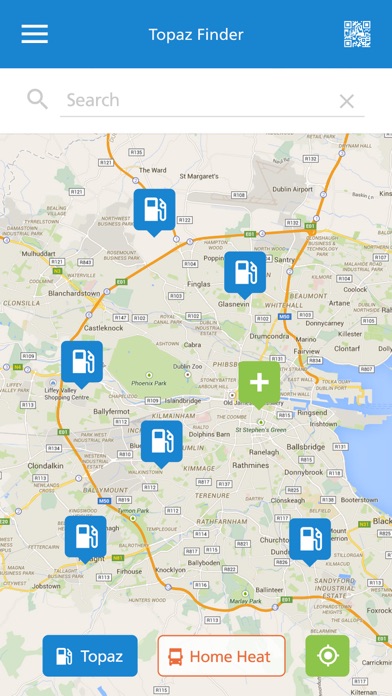This screenshot captures an interface resembling a navigational map application. Dominating the top section is a blue bar displaying "Topaz Finder" in white text at its center. Positioned on the left side of this bar is a menu button, while the right side features a QR code. Directly below lies a white bar extending across the screen, incorporating a search bar. Accompanying the search bar are an X button on its right and a search button on its left. The central portion of the image showcases the map itself, punctuated by six prominent blue square pins and a single green pin. The bottom portion of the screen presents three buttons: a blue button labeled "Topaz," a white button with an orange outline marked "Home Heat" in orange text, and a green square button adorned with a rectangular crosshairs icon.